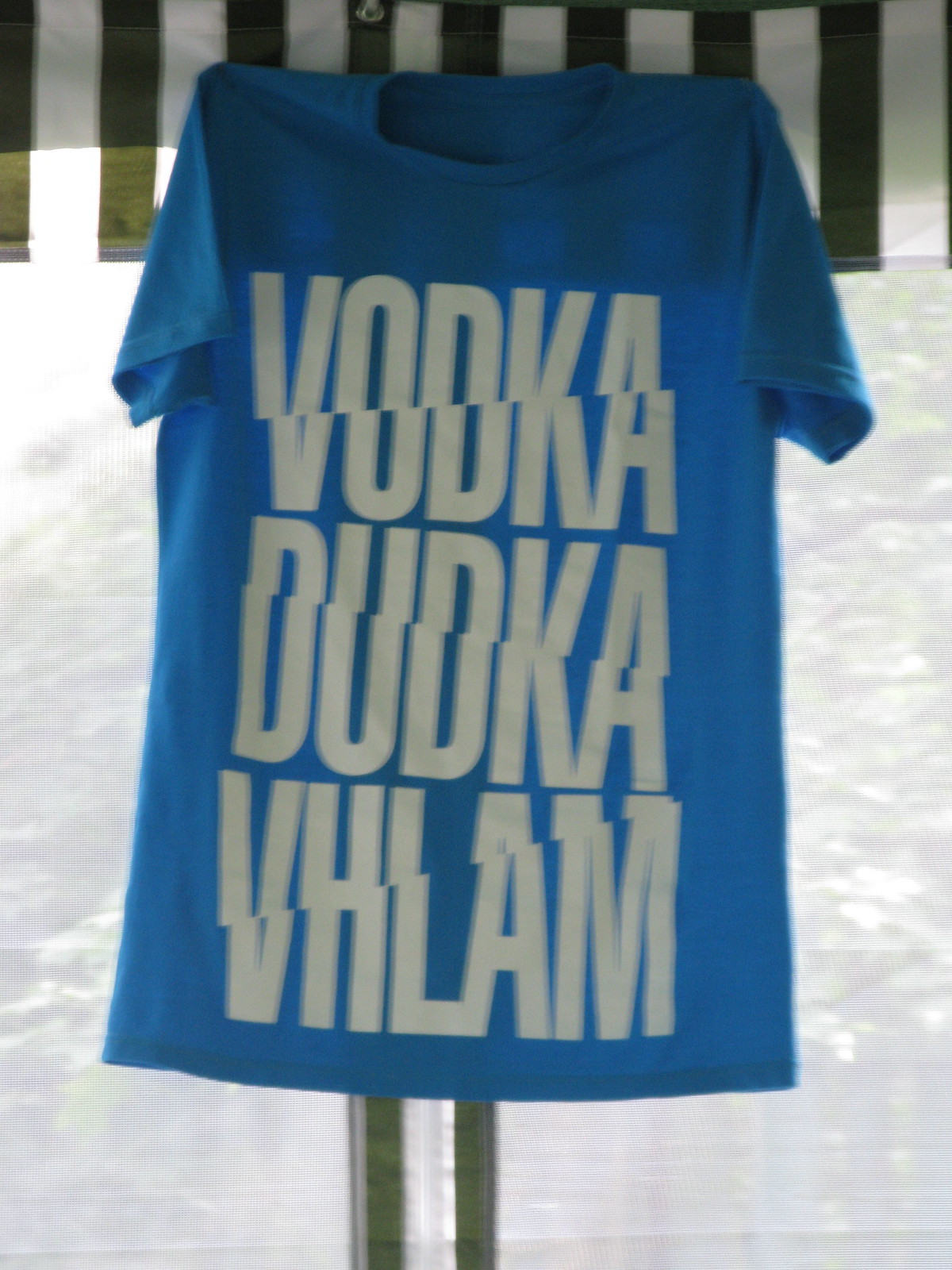This photograph showcases a short-sleeved blue t-shirt hanging on a metal pole. The shirt's fabric is adorned with bold, large white letters printed on its front, which appear to spell out the words "vodka," "dudka," and "vallum." The pole, from which the shirt is suspended, exhibits a dark greenish-gray hue. The background is predominantly white, offering a stark contrast that prominently highlights the t-shirt. While the precise nature of the setting is ambiguous, it could be a bed or possibly a snowy surface. Additionally, at the upper portion of the image, some green and white striped material is visible. The overall composition places the t-shirt as the central focal point against an uncluttered backdrop.